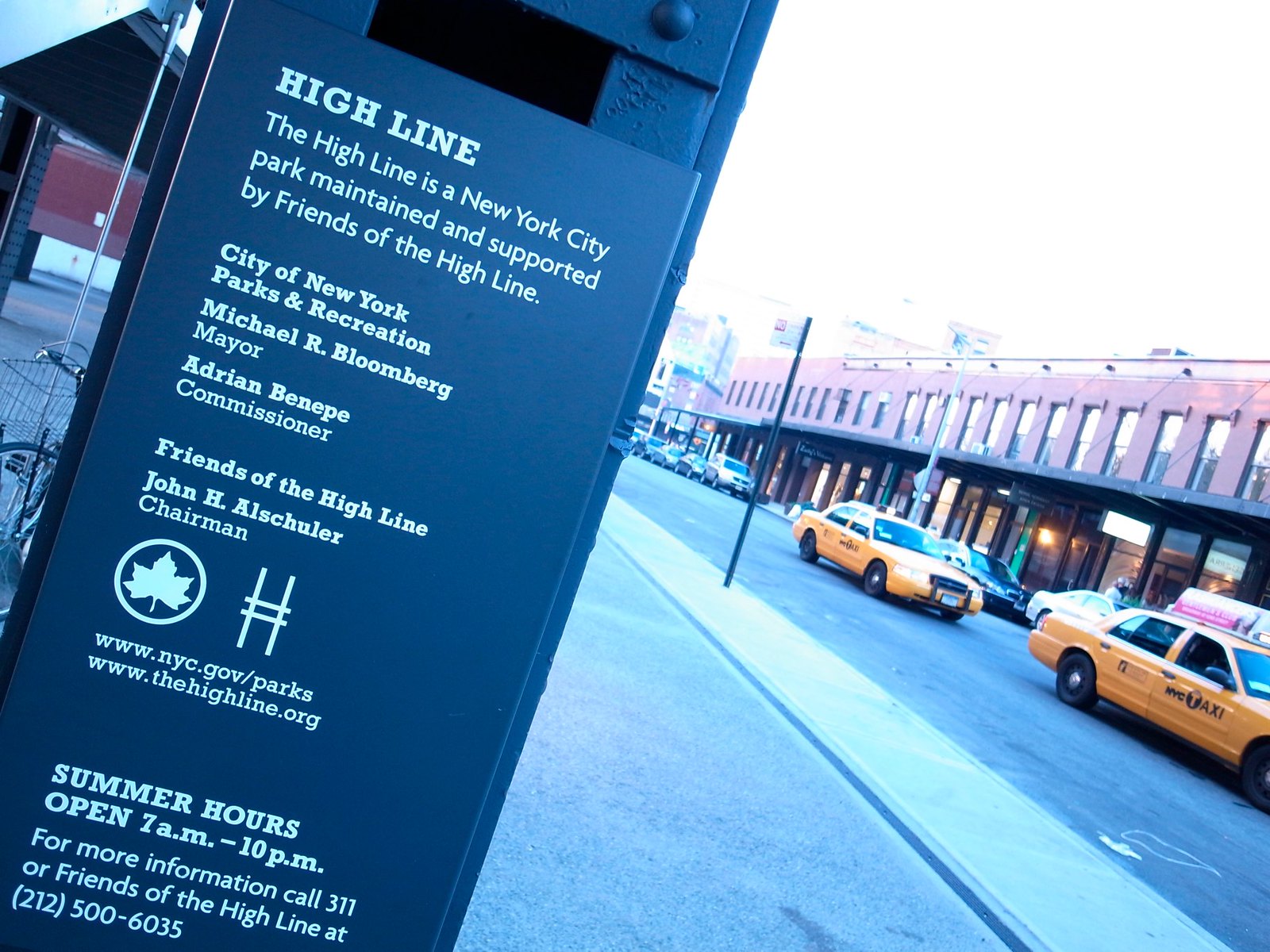This photograph captures a bustling street scene in New York City, with a notable focus on the High Line park. The left side of the image prominently features a detailed blue and white informational sign for the High Line, a park supported by Friends of the High Line, City of New York Parks and Recreation, with names such as Michael R. Bloomberg, Mayor, and Adrienne Benetti, Commissioner, mentioned. The sign includes graphics of a maple leaf and a railroad track, and provides website URLs (www.newyorkcity.gov/parks and www.thehighline.org), summer opening hours (7 a.m. to 10 p.m.), and contact information (Call 3-1-1 or Friends of the High Line at 212-500-6035). Just behind the sign to the left, there's a bicycle rack.

To the right side of the image, a typical city street stretches out with two yellow taxi cabs in motion and several other cars parked along a brick two-story building, suggesting a mix of stores on the lower level and possibly apartments or offices above. The street surface appears to be concrete or asphalt, common for urban environments, hinting at a downtown area. The colors in the photo include blue, white, red, orange, yellow, brown, black, and gray, adding to the midday outdoor ambiance of this New York City scene.